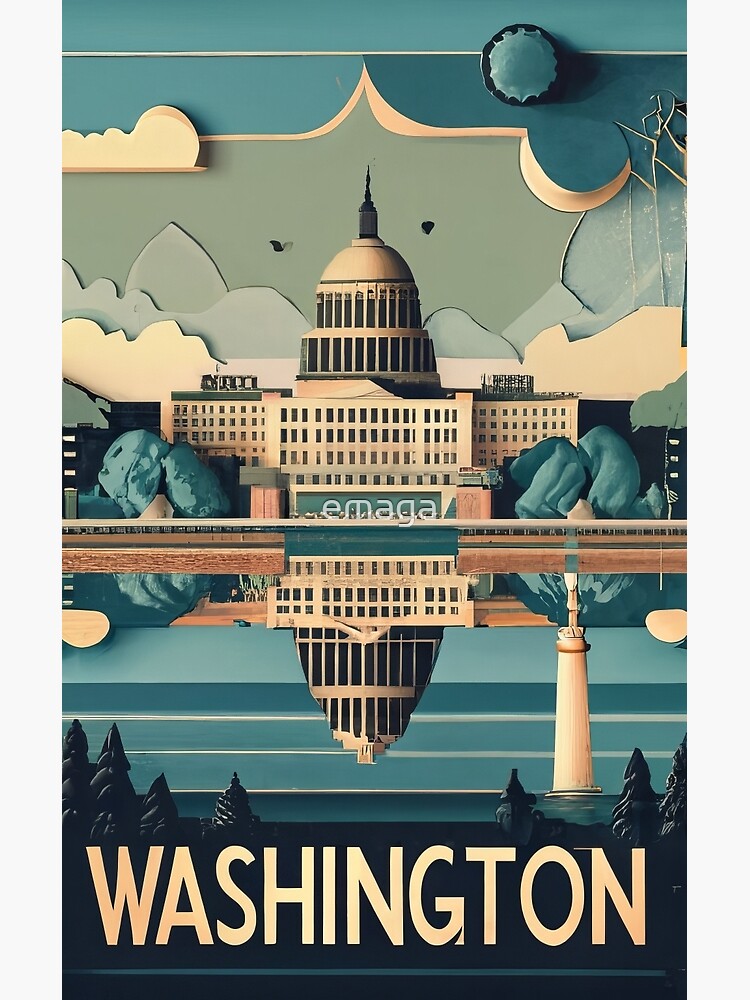This stylized poster in portrait mode features a meticulously crafted depiction of the Capitol building, created using layers of cut-out paper in a digitalized art deco style. The design includes various shapes superimposed to form a detailed image, with the Capitol building prominently displayed and its reflection inverted below, suggesting a serene body of water. The color palette primarily consists of muted tones of teal, beige, and green, with light gray-blue and beige clouds adorning the sky. Grayish-green trees and rolling hills or low mountains form the background elements. Birds are scattered across the sky, adding a dynamic touch to the scene. The word "Washington" is boldly presented in large capital letters at the bottom, lending an unmistakable identity to the composition.